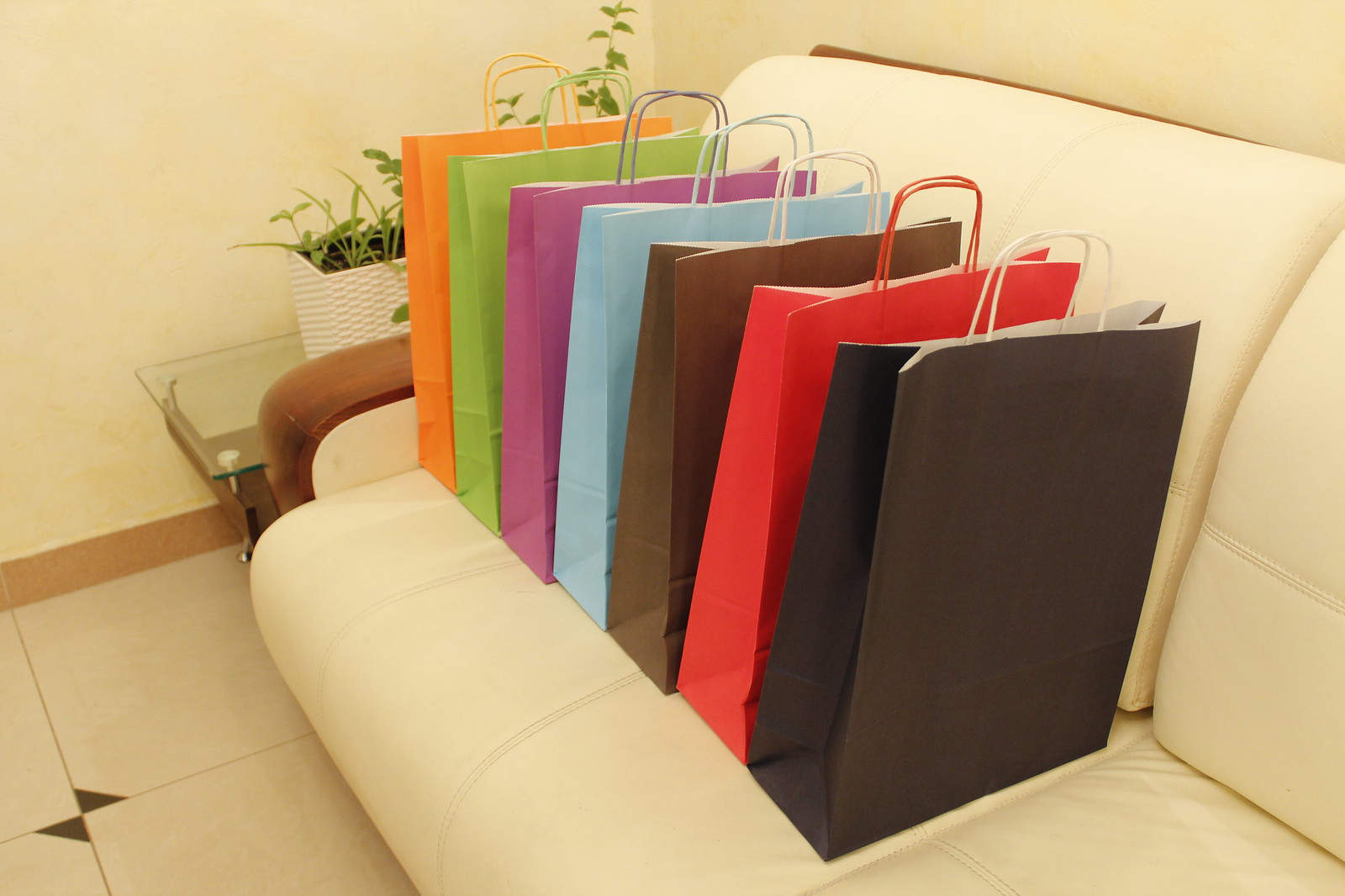The image features a slightly off-white, leather-like couch that resembles car seats, placed within a room that has a clean, somewhat sterile ambiance, similar to a salon or contemporary living space. The room is illuminated with bright, possibly fluorescent, ambient lighting. There is a white or light tan wall adorned with a brown wooden trim at the bottom. The couch sits atop a white tile floor.

Prominently arranged on the couch are seven identically sized and shaped shopping bags, neatly aligned in a row. These bags, which appear to be made of paper and not filled, come in a spectrum of colors: from the back to the front—orange, green, purple, light blue, brown, red, and black.

Near the couch is a small glass end table, upon which sits a white, rectangular ceramic planter holding a green plant. The overall scene is elegantly minimalist, with the multicolored shopping bags adding a vibrant contrast to the predominantly white and neutral-toned setting.